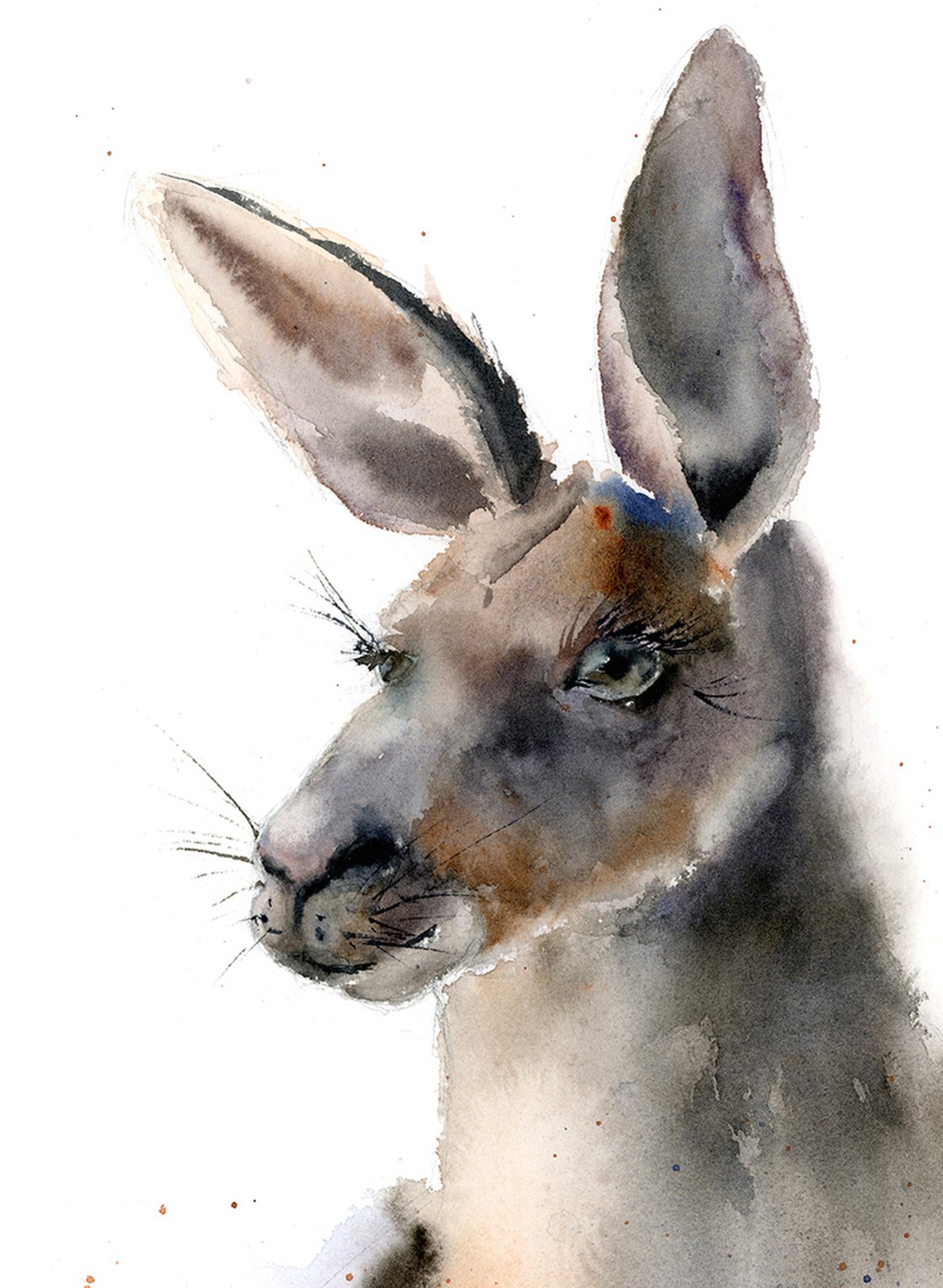This is a detailed watercolour painting of a kangaroo depicted from the neck upwards, focusing on a side profile. The artwork primarily uses various shades of grey, brown, and off-white, with the colors blending softly into one another, creating a pastely effect. The kangaroo’s ears are notably dark grey on the outside, with bits of brown and light grey, and an off-white interior. Its large green eyes with visible black irises and long black eyelashes give it a kindly expression, while its mouth and nose holes are indicated by black color. Long black whiskers extend from its nose, enhancing the intricate details. The kangaroo’s head features patches of brown, and its strong neck is shaded predominantly in grey with hints of off-white and brown. Both ears are portrayed upright, with the right eye only partially visible, emphasizing its left profile. The background is white, further highlighting the delicate and merging colors of the kangaroo, giving it a soft-focus appearance.